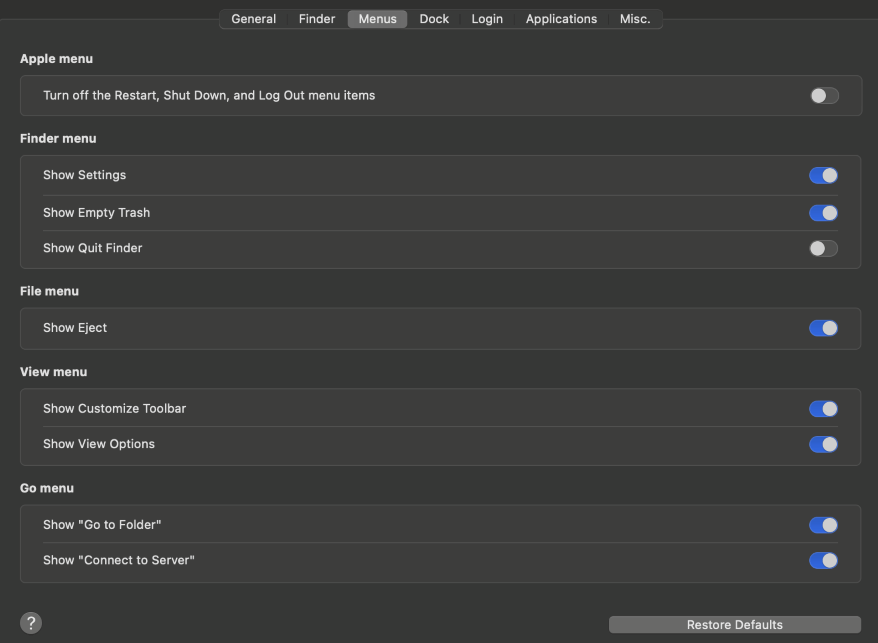A screenshot showcasing a menu interface set in dark mode, featuring a black and dark gray background with white text. At the top of the screen is a horizontally centered menu bar with the following options: General, Finder, Menus, Dock, Login, Applications, and Miss. The "Menus" option is selected, indicated by its light gray highlight. 

On the left side of the page, various menu categories are listed: 

1. **Apple Menu**: Under this category, the option to "Turn off the Restart, Shutdown, and Logout menu items" is present and toggled off.
2. **Finder Menu**: This category includes "Show Settings" and "Show Empty Trash," both toggled on, and "Show Quit Finder," which is toggled off.
3. **File Menu**: Contains the "Show Eject" option, which is toggled on.
4. **View Menu**: Features "Show Customize Toolbar" and "Show View Options," both of which are toggled on.

On the right side of the page are blue toggle switches, indicating active settings. The streamlined design ensures easy navigation and a clear visual hierarchy for user settings.